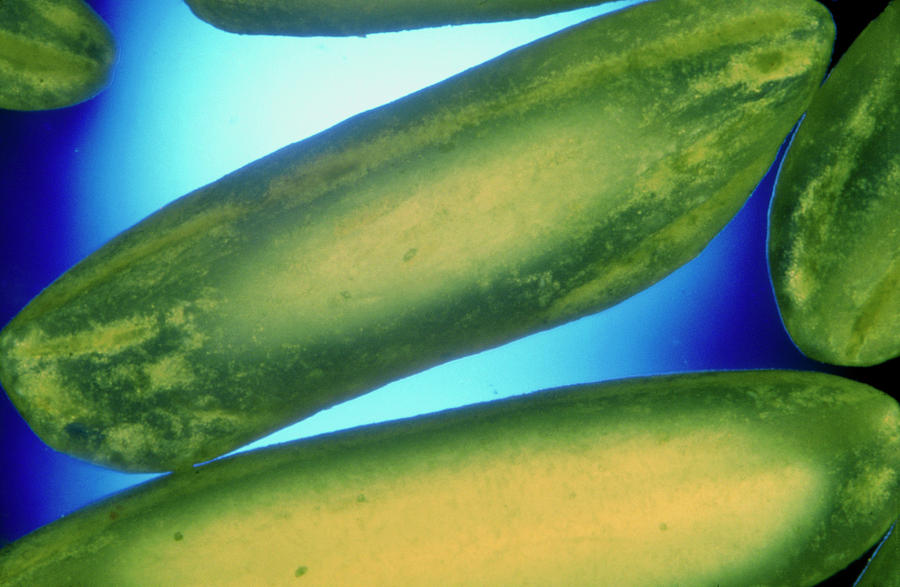This image showcases what appear to be cucumber-like structures set against a gradient blue background. The composition features a wide vertical rectangle format with the background transitioning from a dark blue at the outer edges to nearly white at the center. Scattered across the blue surface are several green, cylindrical objects that closely resemble cucumbers. These objects display a variety of green shades, ranging from dark to light, with some exhibiting yellowish stripes or patches, akin to the undersides of cucumbers. Notably, in the upper left corner, only the tip of one object is visible. A prominently displayed structure runs diagonally from the middle left to the upper right, while another extends from the middle top right downward. Toward the bottom, a longer cucumber-like entity is nearly fully visible, featuring a significant oblong yellow area at its top. The background's hue intensifies to an almost black shade on the extreme right side, further emphasizing the green objects that are dispersed in various angles across the image.